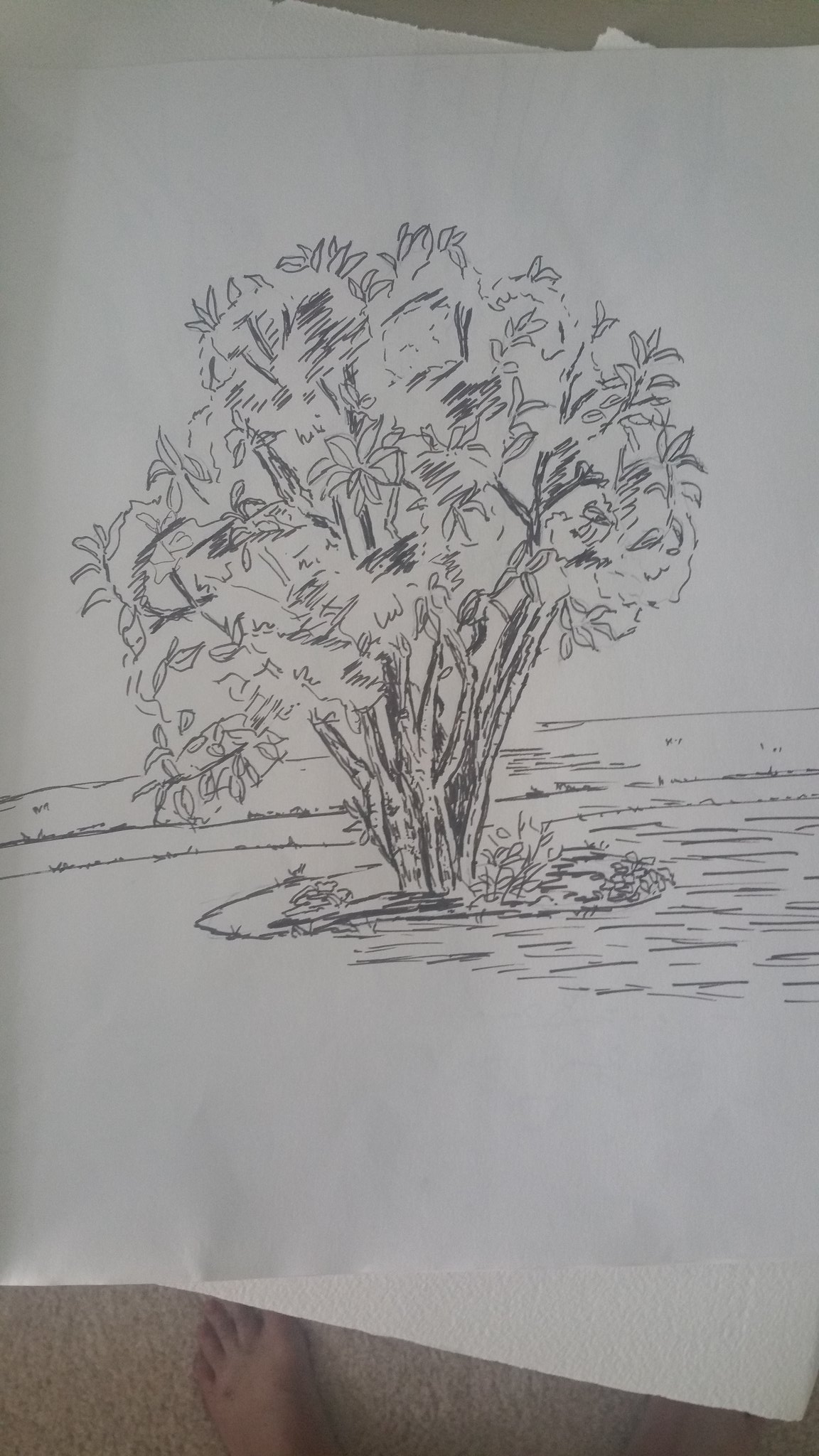This image features an intricately detailed pencil sketch of a tree, rendered on white sketch paper. The tree, positioned centrally on the paper, has a broad, low-hanging structure with numerous branches that extend outward from the ground level. Each branch is adorned with meticulously drawn leaves, indicating the artist's attention to detail. The tree is set against a background that suggests a hilly, grassy landscape, enhancing the naturalistic feel of the drawing. This artwork captures the essence of nature with its careful and deliberate strokes, embodying the serene beauty of a solitary tree in a tranquil setting. No text accompanies the image, allowing the viewer to fully immerse in the visual details and the scene's peaceful ambiance.